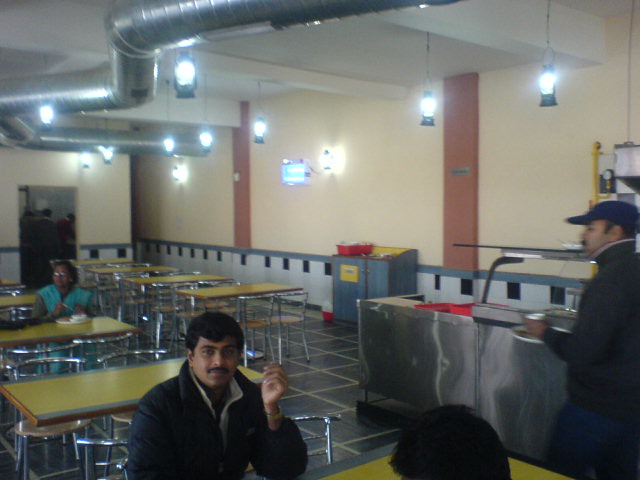This image captures the interior of a bustling cafeteria. The space is adorned with exposed gray ductwork hanging from the ceiling, which also features a mix of recessed lighting and black lantern-like lamps that cast a warm glow. The walls are painted tan with red panels and highlighted by a distinctive blue line that runs across tiles with black squares and white panels.

Rows of rectangular tables with orangish-brown surfaces are paired with steel-framed chairs, each boasting light brown cushions. These simple yet functional furnishings set the scene for the diners. In the foreground, two individuals are seated—one, facing the camera, has dark skin, a simple mustache, short brown hair, and a dark blue shirt or jacket with a white undershirt. He has his right arm raised and a soft smile on his face. His companion, who is closest to the camera, has black hair, the back of their head visible to us. 

To the right, a man clad in a black trench coat and dark blue cap holds a cup in his left hand as he walks past some kind of industrial tray area, possibly for food heating, which adds to the cafeteria's utilitarian ambiance. His distinct facial features include a mustache and sideburns that trail down his ears. Further in the background, a woman with curly brown hair, wearing glasses, a cyan short-sleeved vest, and a long-sleeved gray shirt, sits at another table. Additionally, individuals in an open doorway can be seen peering downwards, engrossed in something unseen.